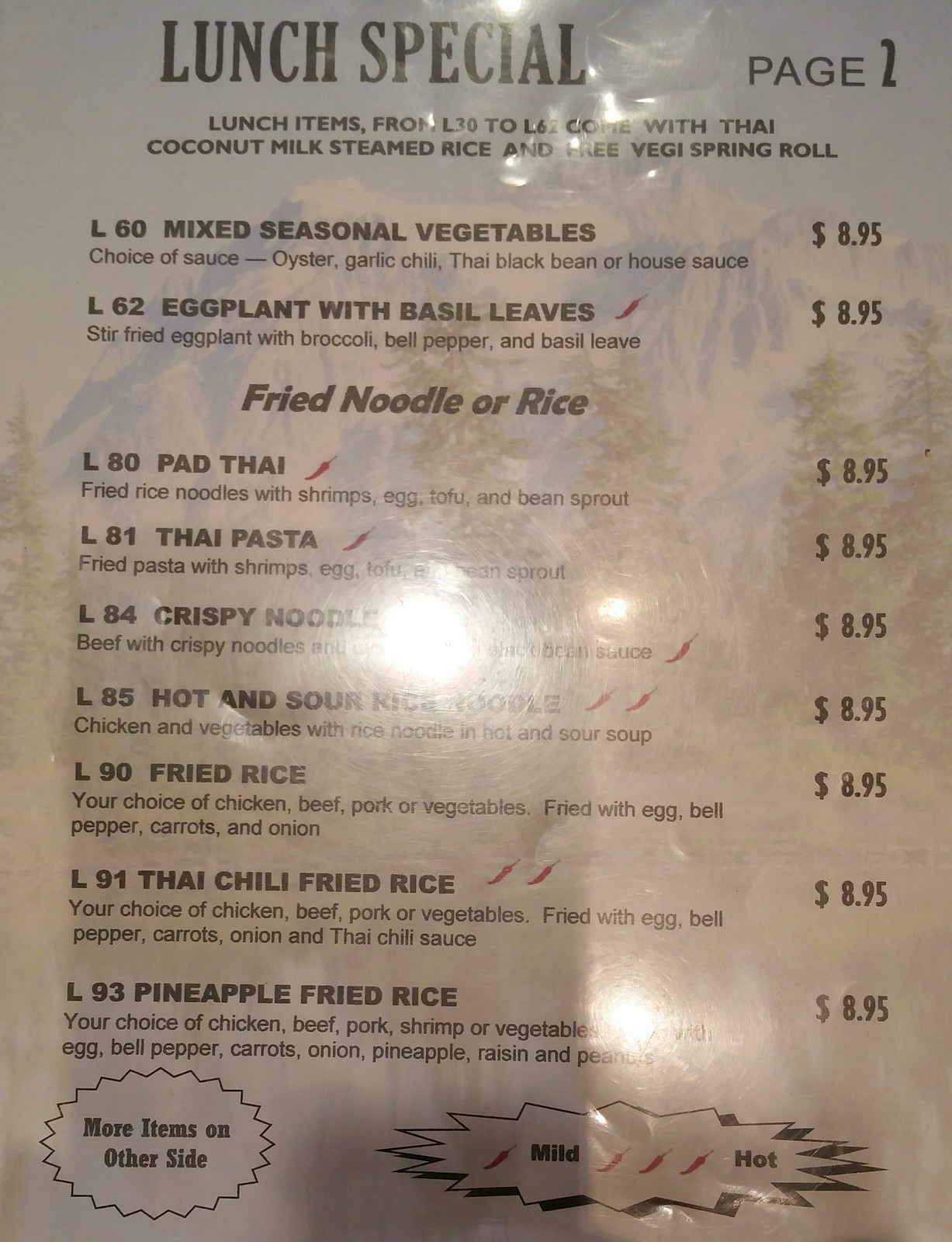Here is a cleaned-up and detailed caption for the image of the menu:

---

This photograph captures a menu from a restaurant, featuring a predominantly white background overlaid with a scenic image of snowy mountains and evergreen trees. The menu has a few bright spots where the lighting reflects, making some areas slightly less visible. At the top, the menu is titled "Lunch Special - Page 1." It notes that lunch items from L30 to L62 include Thai coconut milk, steamed rice, and a free veggie spring roll.

- **L60: Mixed Seasoned Vegetables** - A choice of sauces: oyster, garlic, chili, Thai black bean, or house sauce. Price: $8.95.
- **L62: Eggplant with Basil Leaves** - Stir-fried eggplant with broccoli, bell pepper, and basil leaves. Price: $8.95.

Under the section for fried noodles or rice:
- **L80: Pad Thai** - Fried rice noodles with shrimp, egg, tofu, and bean sprout. Price: $8.95.
- **L81: Thai Pasta** - Price: $8.95.
- **L84: Crispy Noodle** - Price: $8.95.
- **L85: Hot and Sour Rice Noodle** - Price: $8.95.

(Descriptions for items L81 to L85 were less visible due to lighting reflection).

- **L90: Fried Rice** - Your choice of chicken, beef, pork, or vegetables fried with egg, bell pepper, carrots, and onion. Price: $8.95.
- **L91: Thai Chili Fried Rice** - Your choice of chicken, beef, pork, or vegetables fried with egg, bell pepper, carrots, onions, and Thai chili sauce. Price: $8.95.
- **L93: Pineapple Fried Rice** - Your choice of chicken, beef, pork, shrimp, or vegetables, with egg, bell pepper, carrots, onions, pineapple, raisins, and peanuts. Price: $8.95.

The menu indicates that more items are available on the other side. Additionally, there is a scale for the spiciness of dishes, ranging from one pepper to three peppers.

---

This detailed caption gives a comprehensive overview of the menu items and the visual elements of the photograph.